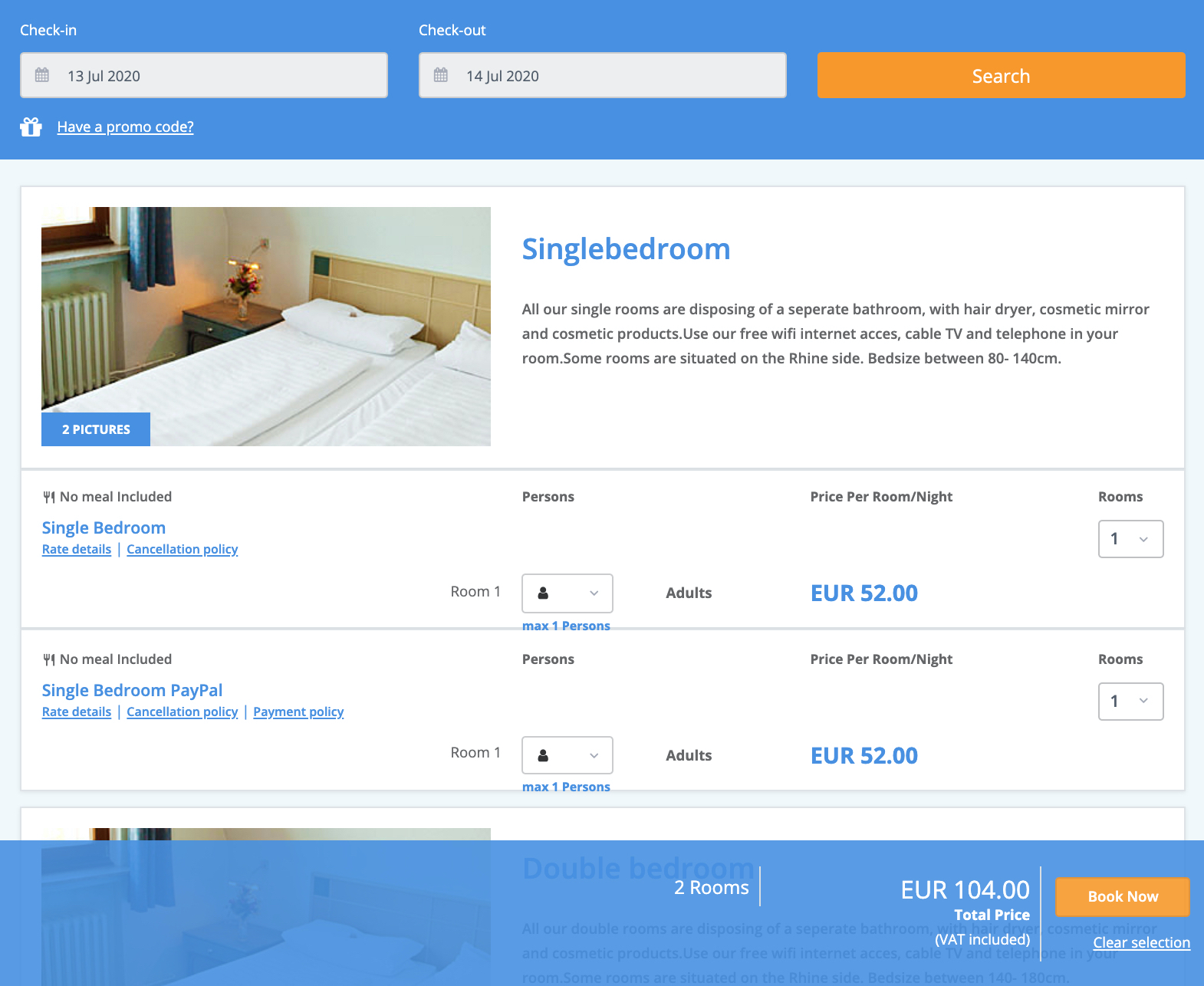This screenshot captures a detailed booking page for accommodation. The website lacks a navigation bar at the top, making it difficult to identify the site at a glance. The page's main body features a white background with a mix of blue and black fonts.

At the top of the page, there is a wide blue banner stretching from left to right. In the top left corner of the banner, a text box labeled "Check-in" displays the date "13 July 2020." Directly beneath, there's a clickable gift icon with the text "Have a promo code?" highlighted. Centrally located within the banner is another text box labeled "Check-out," showing the date "14 July 2020." On the far right of the banner, an orange rectangular button labeled "Search" in white font is prominently displayed.

Below the banner are the search results. The top result features a large photograph on the left side, depicting a bed with neatly folded bedding and pillows, a radiator under a window with two short blue curtains, and a wooden headboard. Adjacent to the photo, the result details a "Single Bedroom," noting that all single rooms come with a separate bathroom equipped with a hairdryer, cosmetic mirror, and cosmetic products. Free Wi-Fi, cable TV, and telephone access are included. Some rooms offer views of the Rhine, with bed sizes ranging between 80 to 140 centimeters. Below these details, a thin blue line separates the information.

Further down, it specifies that no meals are included. The description continues with rate details, cancellation policy, accommodation for one person, at a price of 52 euros per night. Another similar result is listed below, also for a single bedroom, accommodating one person, priced at 52 euros per night.

At the bottom of the screen, there is another wide blue banner. On the far right of this banner is an orange "Book Now" button in white font, with a "Clear Selection" option beneath it. To the left, the total cost of 104 euros is displayed, indicating the booking of two rooms.